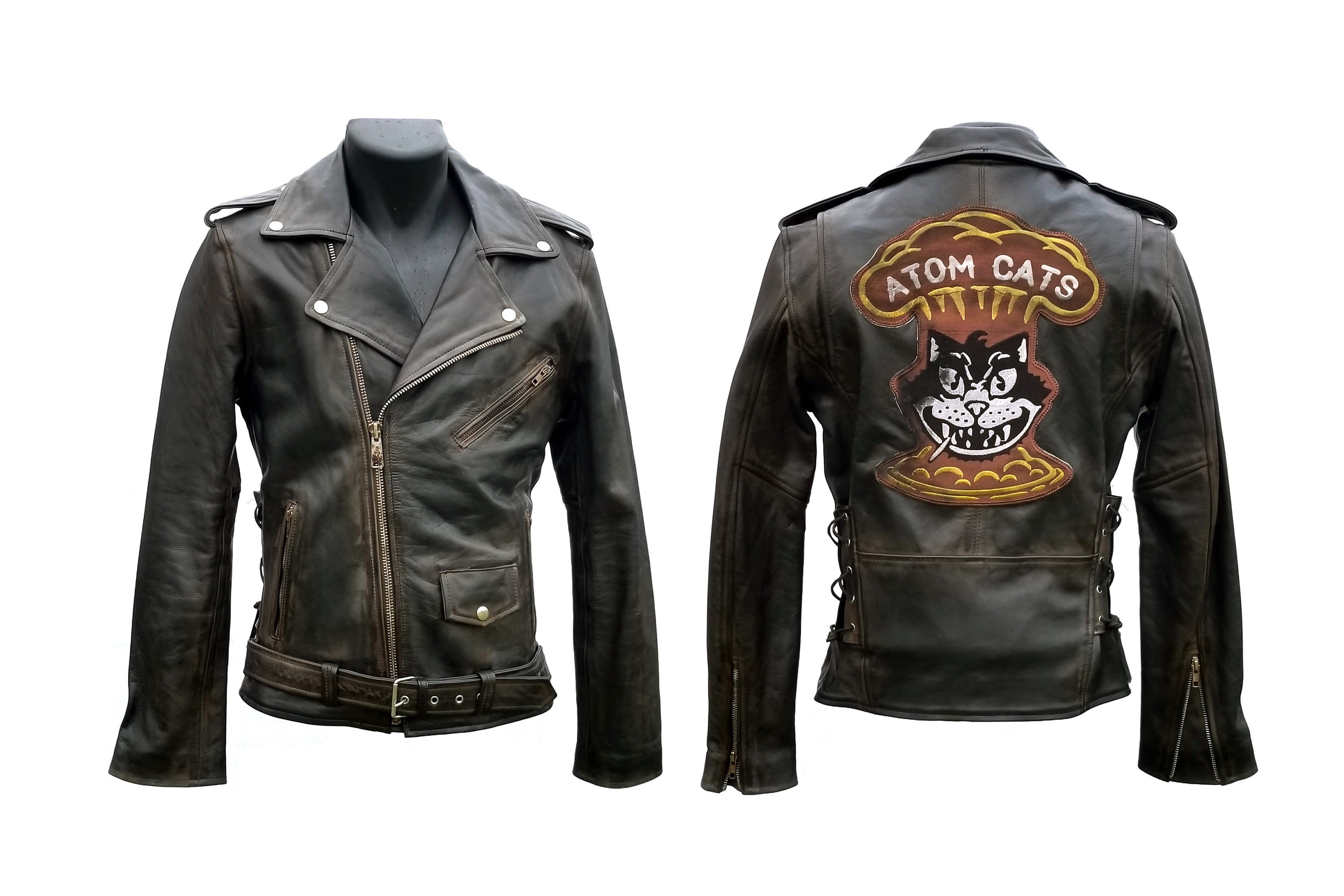This detailed product photograph features both the front and back views of a black leather motorcycle jacket with long sleeves. The front side sports several zippers—including one diagonally placed across the chest and another on a lower side pocket—along with a snap-closure pocket, and a small securing belt just above the bottom hem. The jacket's design includes a belt and some snaps, and it appears to be a stylishly vintage piece, possibly reminiscent of the 1960s.

On the back, dominating the surface is a large, eye-catching patch. This centerpiece depicts a cartoonish cat head with intense, sharp features and a toothpick protruding from its mouth, giving it a mischievous and edgy demeanor. The cat's head is set against a dramatic mushroom cloud, suggesting a powerful explosion. Above and within this cloud, emblazoned in bold letters, is the text "Adam Cats." The combination of the vivid imagery and the text likely signifies a biker group known as the Adam Cats. The jacket, set against a plain white background, emphasizes its role as a classic and visually striking biker gear.